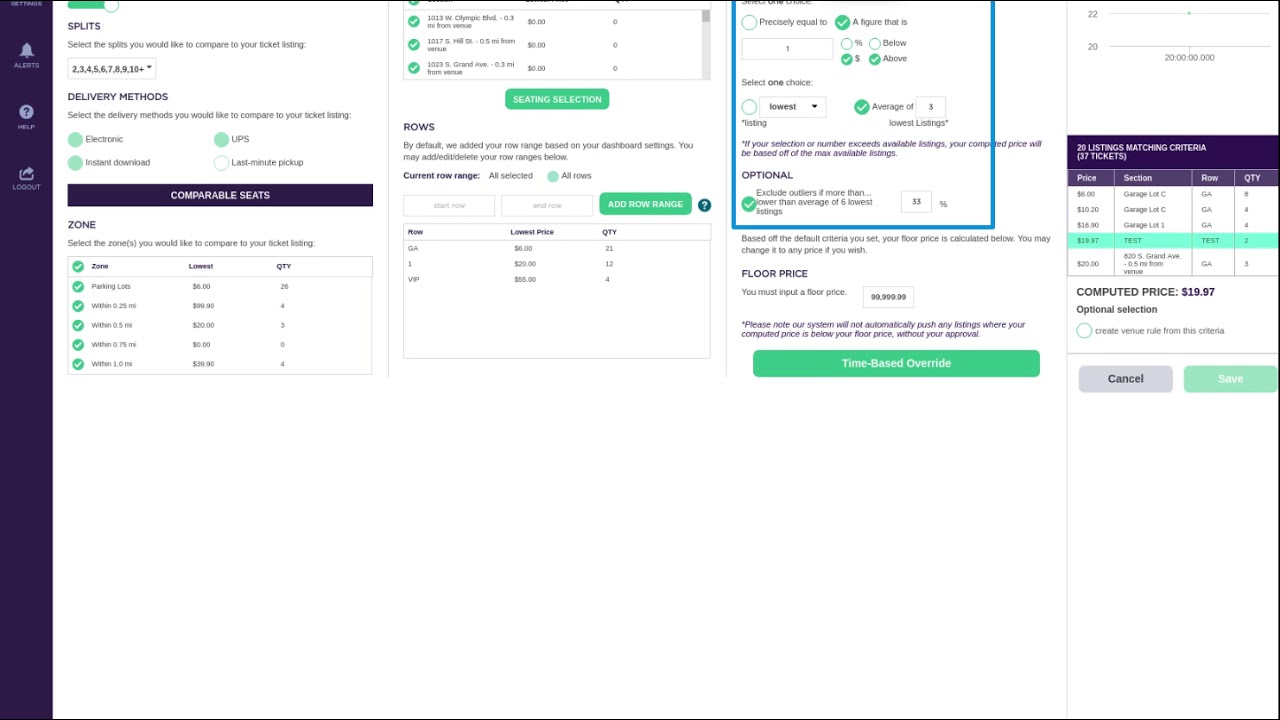This image is a screenshot featuring a user interface with a white background. In the upper left corner, there is a toggle switch, turned on, that has the label "Splits" below it, indicating that the user can select the splits they want to compare to their ticket listing. Below this label, there's a section titled "Delivery Methods," where users can choose from four options: Electronic, Instant Download, UPS, and Last-Minute Pickup.

Following that, there's a black background section with the title "Comparable Seats." Beneath this title is another white area labeled "Zone," where users can select the zone they wish to compare to their ticket listing. The available zones are: Parking Lots Within 0.25 mile, Within 0.5 mile, Within 0.7 mile, and Within 1.0 mile.

In the upper right corner, there's a blue box that reads "Precisely," followed by "Precisely equal to a figure." This area offers options to select a dollar amount with checkboxes labeled "Dollar Sign" and "Above," both of which are checked off.